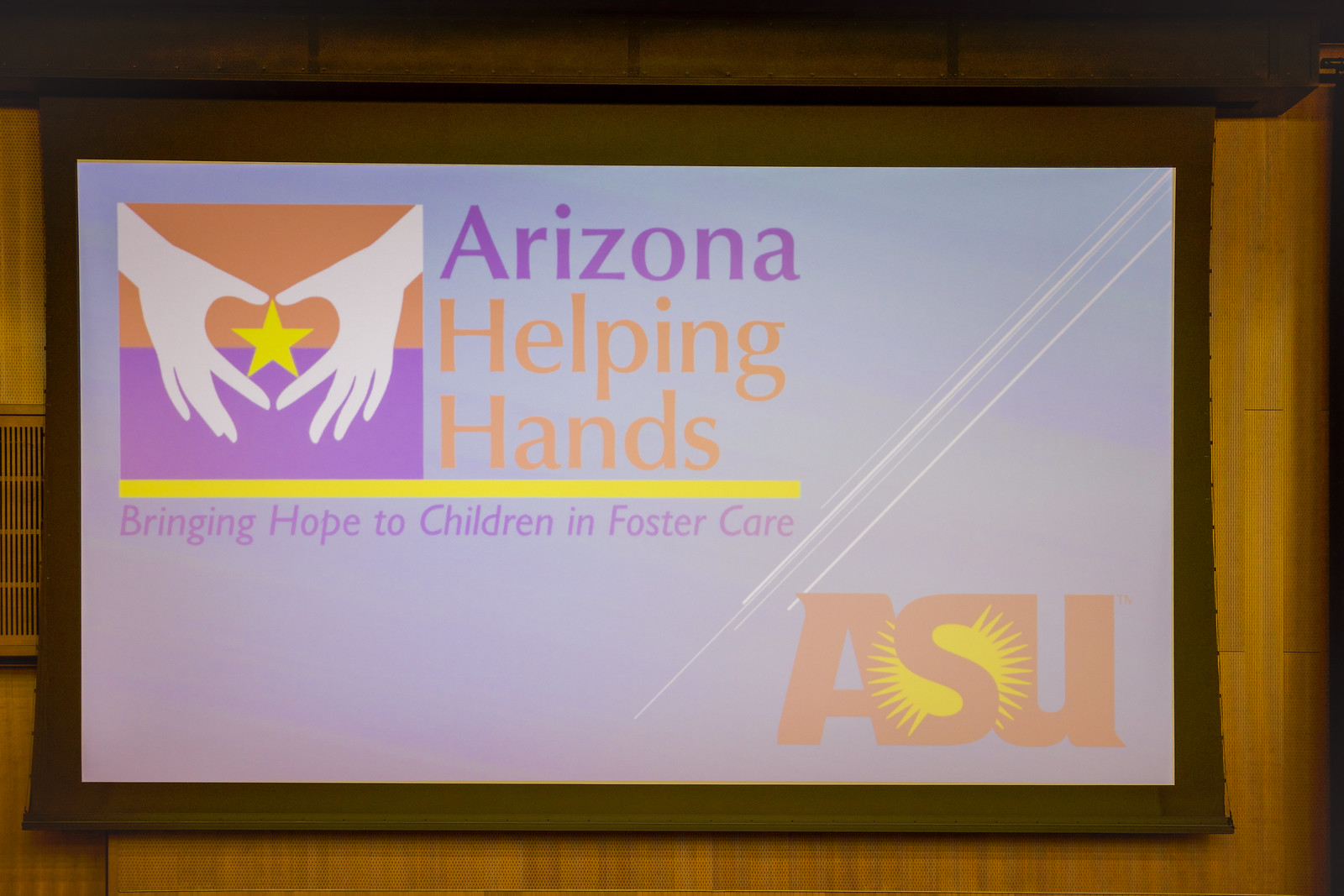This image features a prominently displayed banner with a light purple background. In the top left corner, there is a square composed of an orange stripe and a purple stripe. Within this square, two white hands extend from opposite corners to form a heart, framing a yellow star at the center. To the right of this emblematic square, "Arizona" is written in purple, directly above "Helping Hands" in orange. Below these words and the square, a yellow stripe runs horizontally. Underneath this stripe, in purple font, the slogan reads, "Bringing Hope to Children in Foster Care." Situated in the lower right corner, "ASU" is written in orange with a depiction of a sun behind the letter "S." The banner appears to be hung against a woody, brownish background, resembling a scroll used for projector displays.